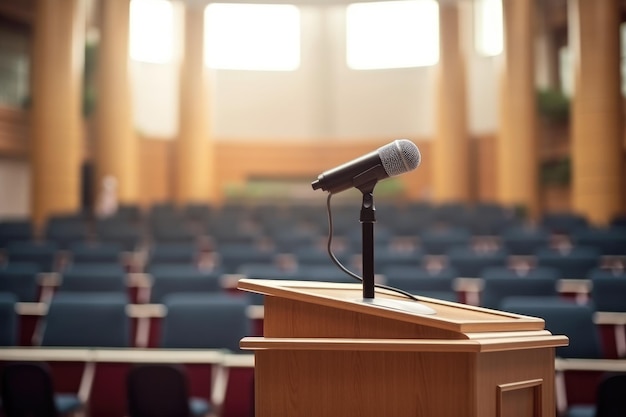The image captures a well-lit auditorium likely set for a conference or lecture. At the forefront, a light brown wooden podium stands with a sleek black and silver microphone perched on top. The background, intentionally blurred, reveals rows of empty blue padded chairs arranged neatly, indicating the anticipation of an audience. Adding to the room's grandeur, six large, orange-yellow pillars stretch up towards the high ceiling, while sunlight streams in through upper windows, enhancing the room's warm and inviting atmosphere. Amidst the blurred details, subtle hints of red peek between the rows of chairs, contributing to the overall color palette of yellows, browns, blacks, and blues. The focused composition emphasizes the podium, highlighting its role as the centerpiece in this spacious and orderly setting.